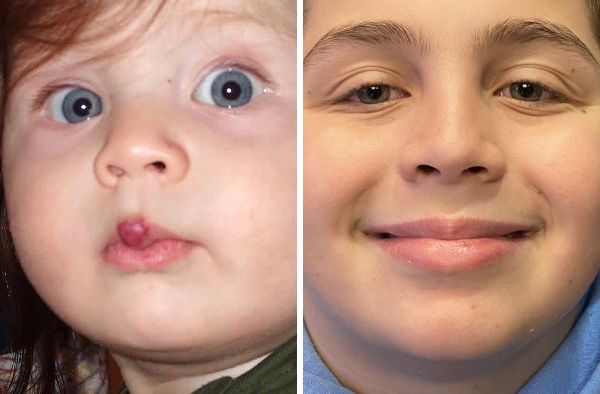The image is a photoshopped side-by-side comparison of two close-up photographs, highlighting a significant transformation. On the left, there's a close-up of a young child, possibly a boy around two to five years old, with distinct features: big, bright blue eyes, long reddish-brown hair with visible bangs, and chubby cheeks. He has a noticeable heart-shaped red mark on his upper lip, suggestive of a cleft palate or similar malformation. This child has a curious and slightly surprised expression, and is wearing a shirt, though only the top is visible.

On the right, the image showcases an older individual, likely in their late 20s, presumed to be the same person but now fully grown. This young man has green or hazel eyes, dark eyebrows, a well-shaped nose, and a broad smile that causes his eyes to squint slightly with happiness. He is seen from the forehead down to his neck, dressed in a blue shirt. His lips appear normal, implying corrective surgery or healing of the previous condition, creating a heartwarming 'before and after' visual narrative.